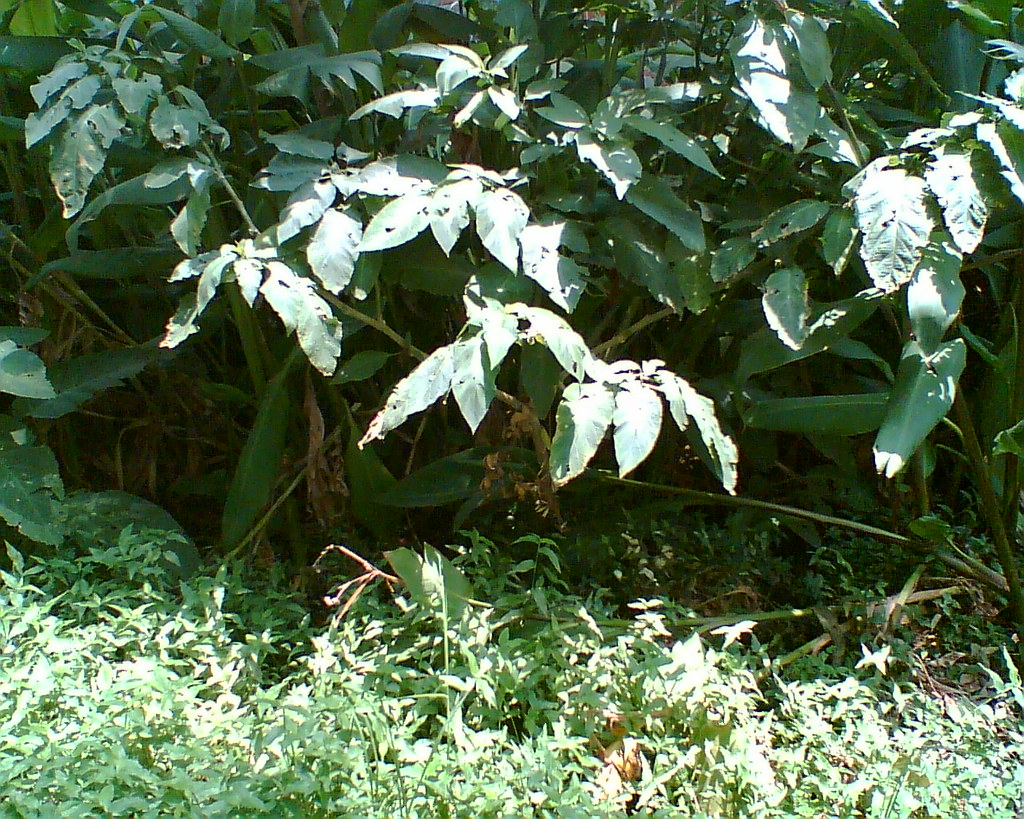This outdoor photograph captures a dense, leafy green area dominated by a sprawling bush with rounded leaves. The bush occupies most of the middle to upper sections of the image and displays a mixture of vibrant green leaves interspersed with some brownish and slightly wilted ones, especially in the shaded areas. Sharp, small ends are observed on several leaves, and a few even have holes, giving them a worn appearance as if they are weathered or have been nibbled by creatures.

In the lower part of the image, clusters of smaller leaves and stems emerge from a bed of lush green grass that reaches up to meet the overhanging foliage of the bush. A notable play of sunlight filters through, casting bright highlights on some leaves, making them appear almost white, while others are left in the shadows, creating a darker green contrast. The bright sunlight is predominant and seems to come from the right side, illuminating parts of the bush and causing glare, while leaving the undersides and inner sections shrouded in a cool shade. There are no human elements or other distractions in this natural scene, emphasizing the dense greenery and intricate interplay of sunlight and shadow.